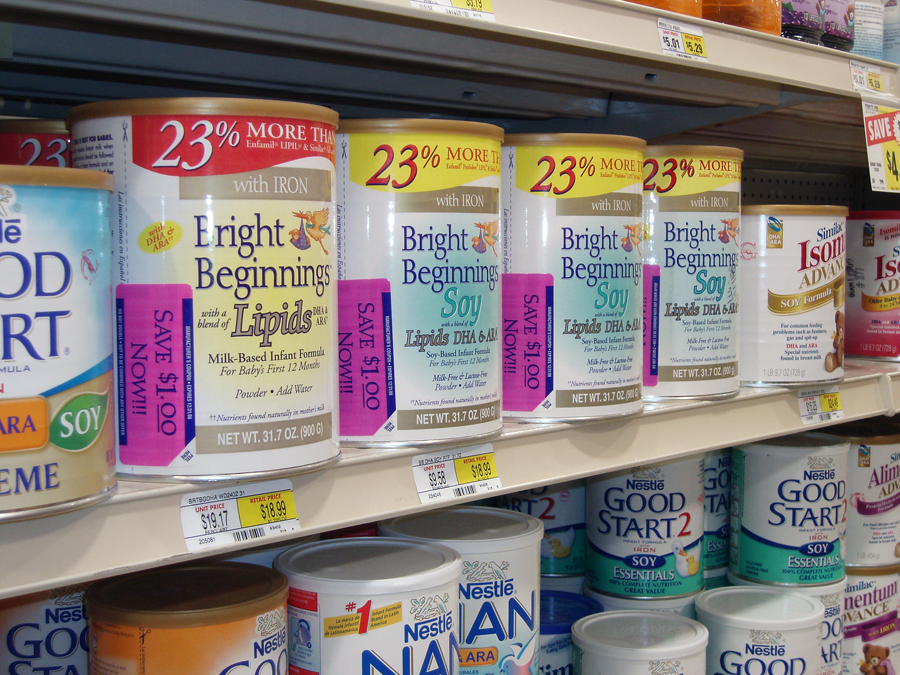In this rectangular image, we are presented with a section of store shelving dedicated to baby formula. Set against tan metal shelves, the focus is on an assortment of formula cans. The central shelf prominently displays these items, while the lower shelf is partially visible, giving a glimpse of more products. 

From left to right, the first item is a canister of Bright Beginnings Milk-Based Infant Formula, distinguished by its white body and gold lid. Attached to the left side of this can is a purple, peel-off coupon with the text "Save $1 now." Four cans of this Bright Beginnings formula are lined up side by side. 

At the far right end of this row, we find a smaller can of Similac Advance Soy Formula, distinctively smaller in size compared to the Bright Beginnings cans. Below these products, the tops of additional baby formula containers are visible, including a can of Nestlé Good Start, recognizable by its white and mint green design. 

This image captures a snapshot of the variety and organization within the baby formula section of this store.